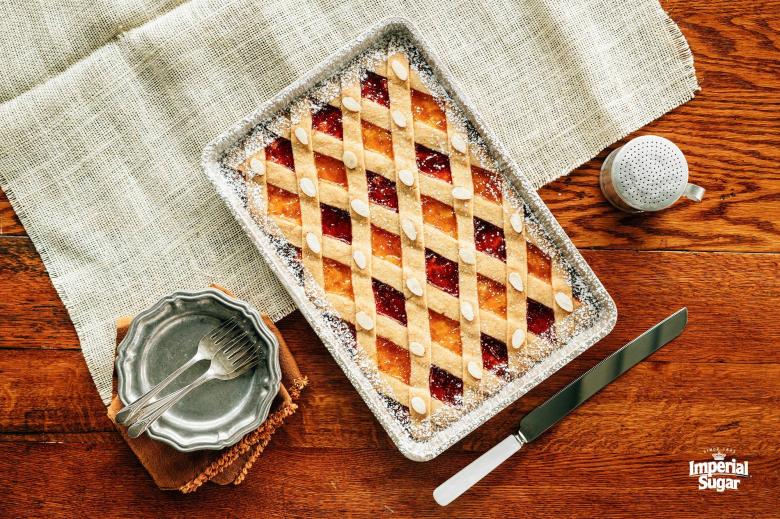This advertisement photograph for Imperial Sugar showcases a delectable rectangular fruit pie with a lattice crust, alternately filled with vibrant red cherries and orange peaches. The pie, placed in a 12x18-inch baking dish, is adorned with white decorative dots at each lattice intersection and a dusting of powdered sugar around the edges, highlighting its golden-brown finish. The setting, a rustic wooden table, features a partially spread gray linen cloth, enhancing the homemade appeal. Accompanying the pie, a white-handled stainless steel slicing knife rests to the right, alongside a silver powdered sugar shaker. To the left, a stainless steel dish containing three forks sits atop a folded brown cloth napkin. The bottom right corner of the image bears the Imperial Sugar logo in white font, cementing the brand's role in this culinary creation.